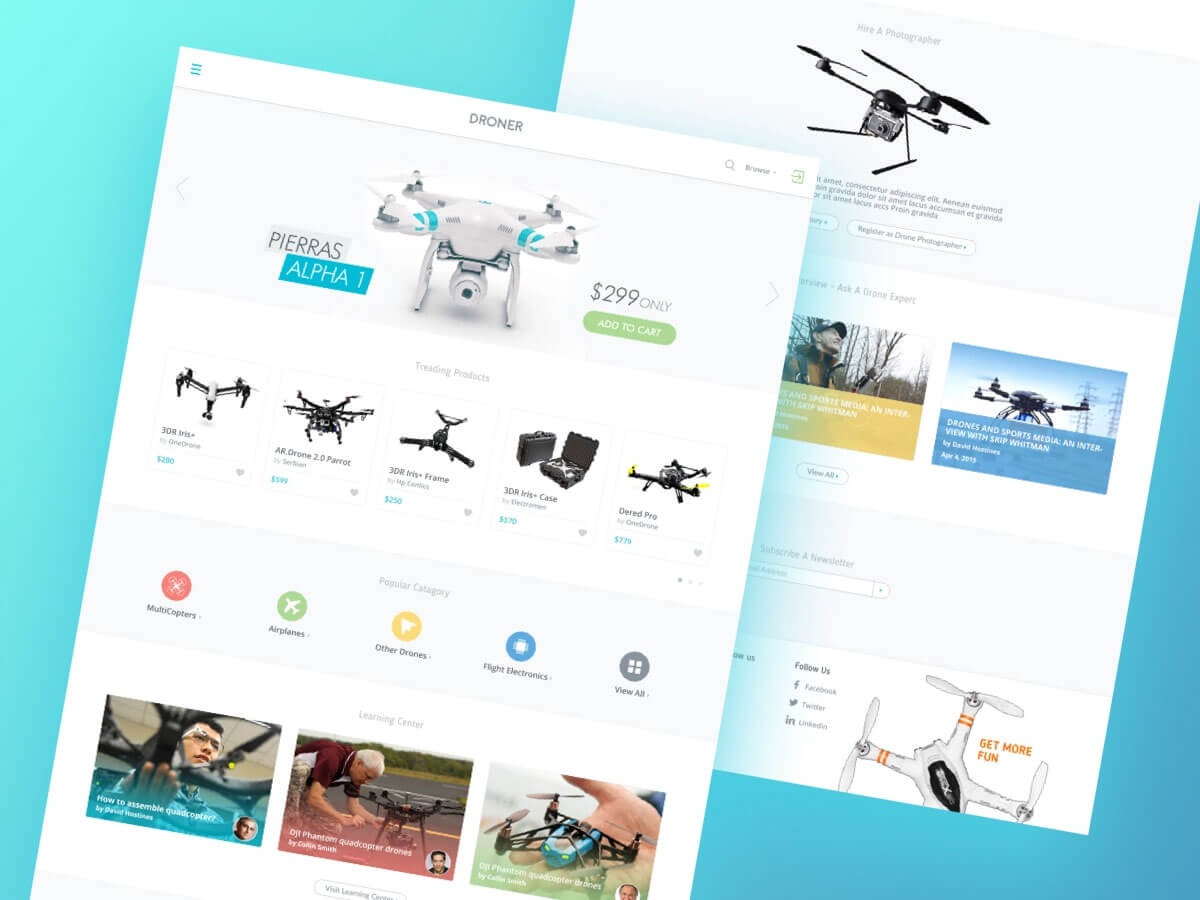Here is a detailed and cleaned-up caption for the image described:

---

The image features a section of a website named "Droner," which has a turquoise background. The webpage displays two slightly angled white pages, skewed from the bottom left to the top right but at a gentle incline.

The first page prominently displays the word "Droner" and features a product listing for drones. At the top of this page, there is a highlighted product named "Pierras Alpha One," priced at $299 with an "Add to Cart" button below it. Below this section, there is a row listing five different drones, each accompanied by their names and prices, although the details are somewhat difficult to read.

Underneath the drone listings, there is a navigation menu with categories, which likely include "Multi Copters," "Airplanes," "Other Drones," "Flight Electronics," and "View All." Below this, a row of three photos is partially visible, with the text being mostly illegible.

The second page in the background showcases a drone image where all its individual parts are laid out meticulously. Below this image, there are three additional photos, though the specific details remain unclear. The overall color scheme of the website encompasses turquoise, blue, red, yellow, green, gray, and white.

---

This caption provides a clear, structured, and detailed description of the image content.